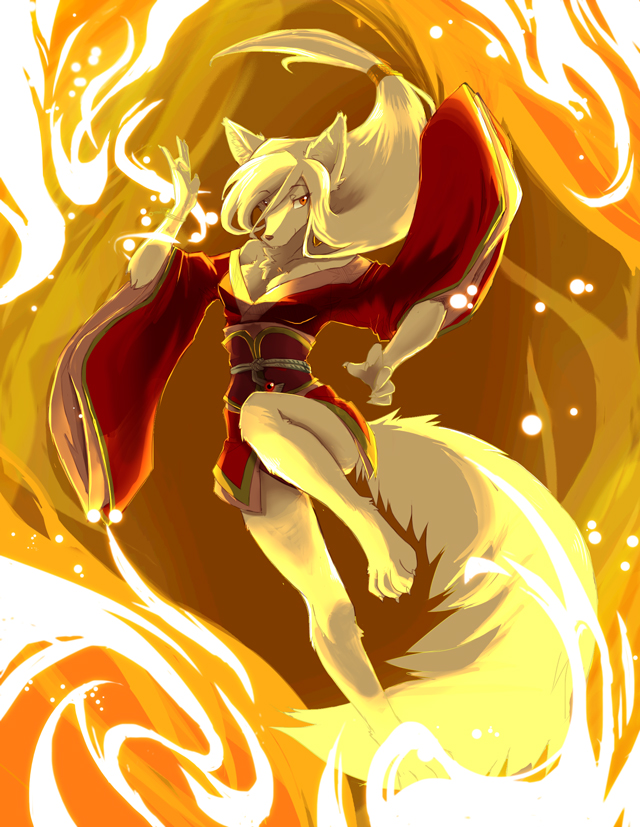This detailed, vibrant artwork likely represents fan art, possibly inspired by anime. The piece is a vertically rectangular painting awash in swirly hues of oranges, reds, yellows, whites, and golds, creating a fiery impression. Central to the image is a striking female figure with the head of a dog or wolf, adorned with long, flowing white hair and ears, and a long, fluffy, white tail. The character is dressed in a distinctive, short red silk dress with massive, flowing sleeves. The intricate details of her human-like female form are emphasized by her curvy figure, bare legs, and feet. The dynamic pose shows her jumping or possibly marching with one foot raised, one hand bent at the elbow pointing upward, and the other hand reaching toward the viewer. Enhancing the sense of movement and energy around her, the background swirls in colors that resemble flames.